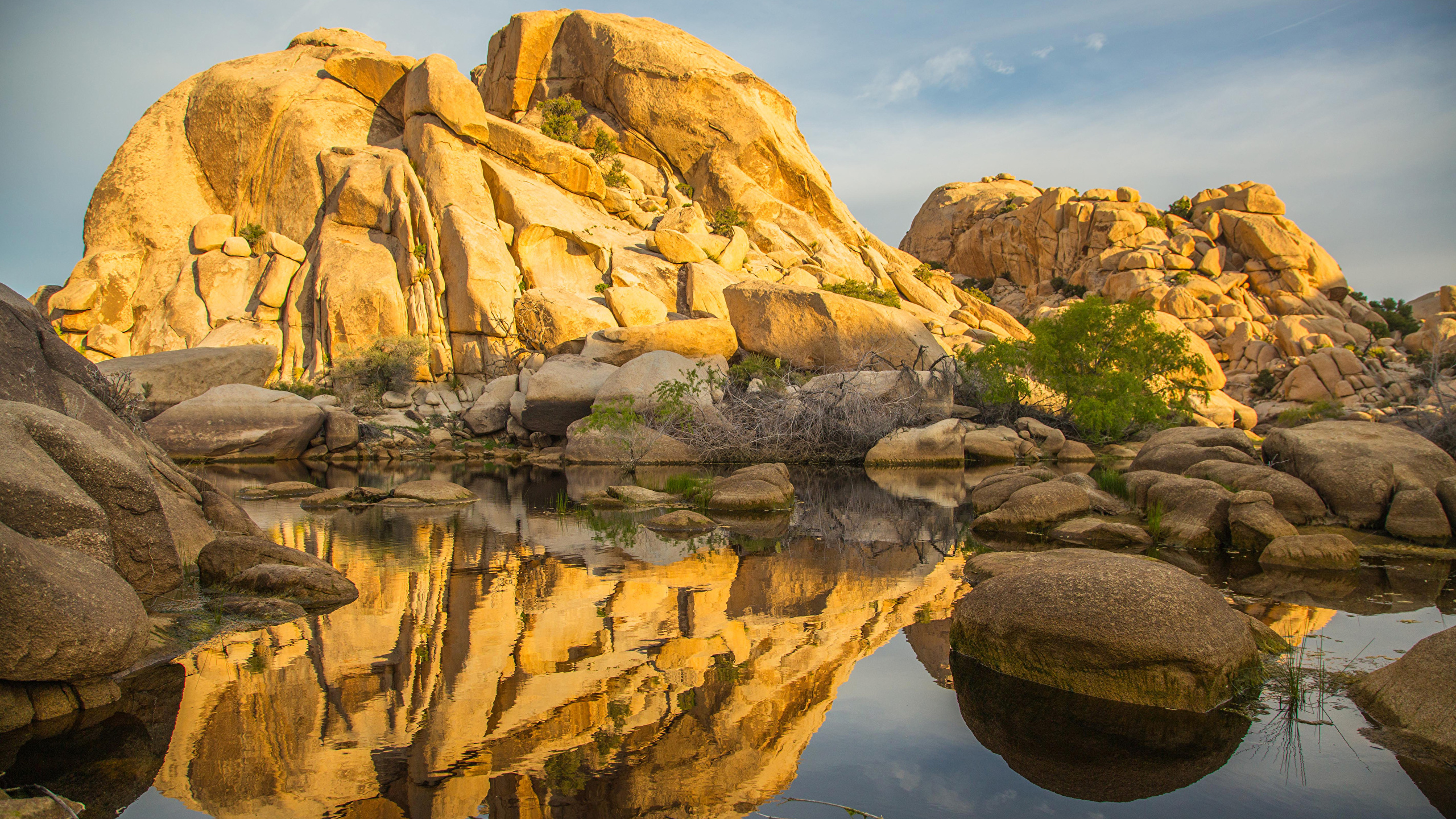The photograph captures an extraordinarily pristine, outdoor natural setting that evokes a sense of untouched serenity. Dominating the bottom half of the image is a small, calm water body or lake, its surface still and reflective. Surrounding the water body are large, dark brown boulder-type rocks, both along the shoreline and within the water itself. These rocks have a dark beige tone, contrasting with the yellowish-tan hue of the large craggy rock hill that rises prominently in the upper left of the image. This hill, composed entirely of rocks and stones, appears almost golden in the sunlight and features patches of green plants. To the right of this imposing formation is a smaller, similar rocky hill. The azure blue sky above, with its few scattered clouds, mirrors itself perfectly in the tranquil surface of the lake, creating an almost surreal, symmetrical reflection. Framing the scene, small green plants with branches and tiny trees add a touch of verdant life, making the entire composition look almost too pristine, as if crafted on a sound stage.